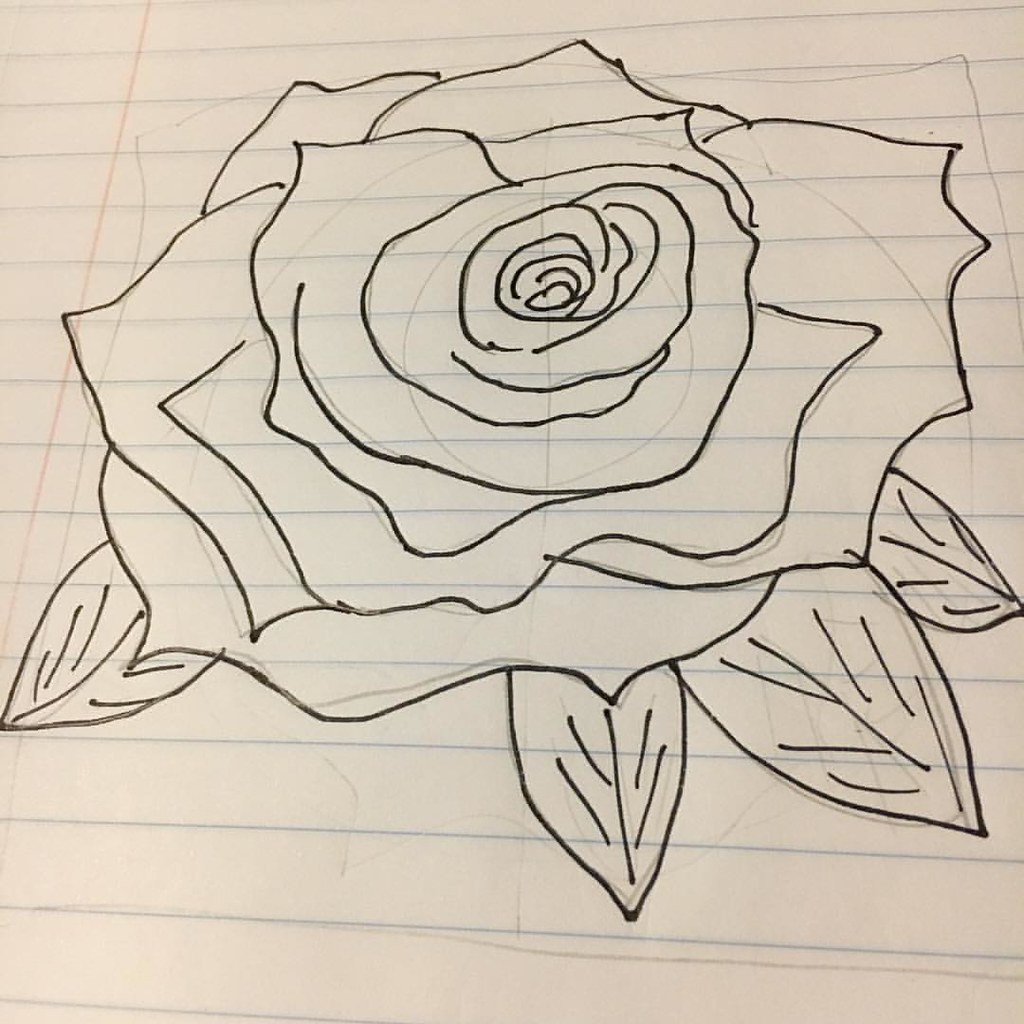This is a detailed sketch of a fully-bloomed rose, drawn in black marker on lined loose leaf notebook paper. The paper's horizontal blue lines and the light reddish left margin line are visible, although the image is zoomed in to primarily focus on the rose sketch itself, making the edges of the paper out of frame. The sketch appears to have been first lightly outlined in pencil, with visible faint graphite marks suggesting an initial draft that was traced over. The entire drawing is in black, with no additional color, and it consists of a large, detailed rose that nearly fills the entire image frame, extending almost to the left, right, and upper borders. The rose is depicted in a simple style, showing petals and leaves with identifiable veins. There are four pointed leaves, each oriented in specific directions: one towards the lower left edge, another straight down the center, a third toward the lower right edge, and the fourth to the middle of the right side. Each leaf is drawn with distinct vein lines, giving a V-shape appearance with detailed black lines.